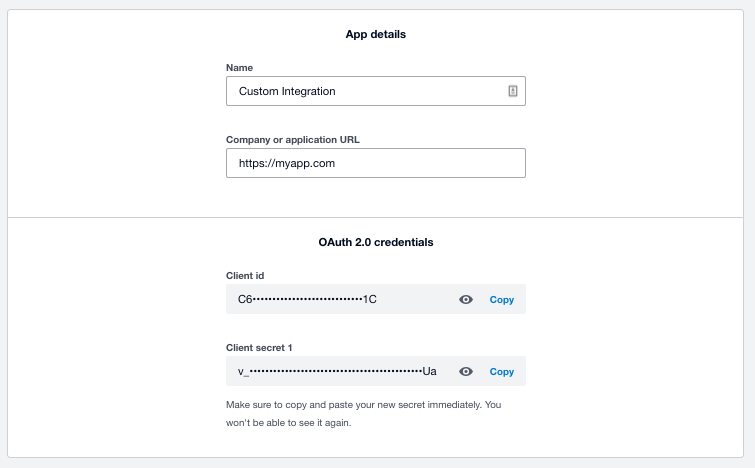The image depicts a form page split into two sections by a gray horizontal line. 

In the top section, the heading "App Details" is shown in bold black text. Below this, the label "Name" appears, followed by a text box that contains the text "Custom Integration" in black. Adjacent to this text box, there is a small symbol.

Following that, the label "Company or Application URL" is visible, with another text box below it. This text box contains the URL "https://myapp.com."

Below the horizontal line, the heading "OAuth 2.0 Credentials" is also in bold black text. The label "Client ID" is seen next, accompanied by a text box with partially obscured text: "C6********1C". There is an eye symbol next to this text box for users to click on to reveal the entire client ID and a blue "Copy" link on the right.

Further down, the label "Client Secret" is displayed, followed by a text box containing "V_******UA". This section also includes an eye symbol for revealing the secret and a blue "Copy" link. At the bottom of this section, a note reads: "Make sure to copy and paste your new secret immediately. You won't be able to see it again."